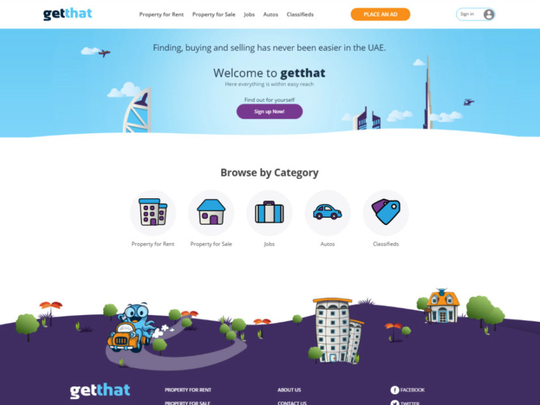**Website Overview: Get That**

The homepage of the Get That website, dedicated to users in the United Arab Emirates (UAE), features the company logo prominently in the upper left-hand corner. The logo “getthat” is written in a small, lowercase font with "get" in dark navy blue and "that" in a light sky blue, all run together without spaces.

At the top of the website, a substantial banner states, “Finding, Buying, and Selling has never been easier in the UAE,” setting the tone for the site’s purpose. Just beneath this header, a welcoming message, “Welcome to Get That,” is displayed adjacent to a prominent purple button inviting users to “Sign Up Now.”

The site adopts a clean, minimalist design with a white background. Centrally positioned on the page, the text “Browse by Category” is printed in bold black letters, serving as a guide to the various offerings of the site. These categories include:

- **Property for Rent:** Represented by an icon of an apartment building.
- **Property for Sale:** Illustrated with a small house icon.
- **Jobs:** Denoted by a briefcase icon.
- **Autos:** Marked by a blue car icon.
- **Classified:** Shown with price tags icon.

Below these categories, the website features a picturesque suburban scene. The unique graphics include a dark purple ground and a winding light purple road, along which an orange car is driving by. This area is interspersed with trees, contributing to a serene suburban vibe.

Overall, the neatly arranged icons and descriptions help guide users seamlessly through the process of finding, buying, and selling in the UAE.